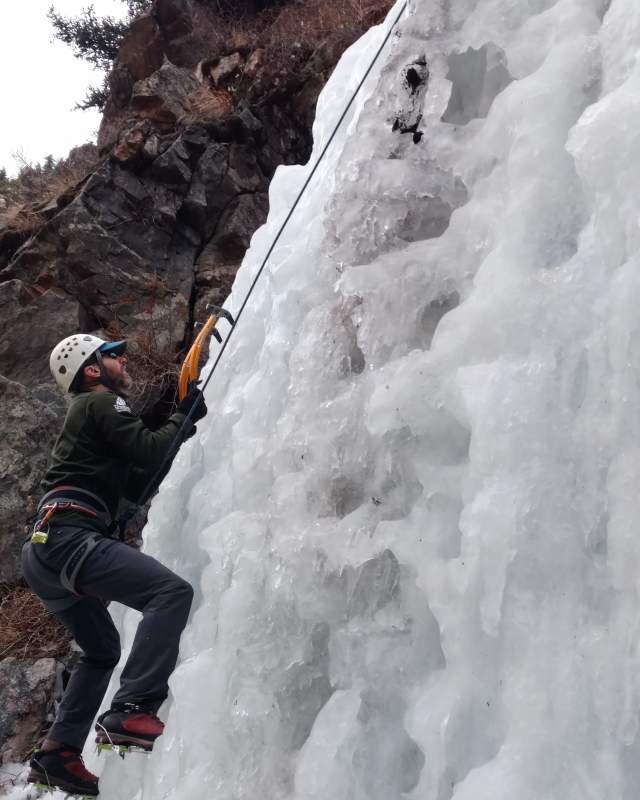The color photograph captures a man in mid-climb on a frozen ice wall outdoors during the day, utilizing natural light. The subject, situated in the bottom left of the vertically rectangular image, wears black long pants, red and black shoes equipped with green metal cleats, and a black and red harness. His upper attire includes a long-sleeve green felt jacket, black gloves, and a white safety helmet, beneath which he sports sunglasses and a short brown beard. He is climbing with the aid of blue and orange-handled ice picks with black curved heads, gripping the ice wall. His harness is connected to a black rope secured to a higher point. In the background, a gray and black cliff wall covered with sparse vegetation stretches upwards. A section of dark brown rock outcropping is visible to the left, adorned with small patches of green plants. The overall composition captures the realism and adventurous intensity of the scene.